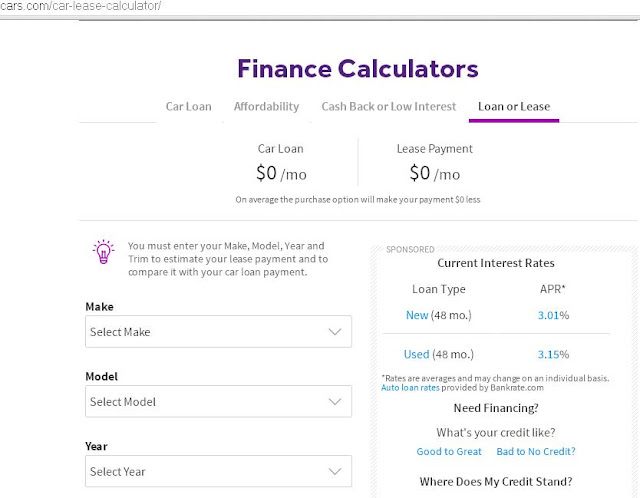This is a screenshot from the Cars.com website, specifically from its Car Lease Calculator page. The website background is white, and the page title "Finance Calculators" is displayed in a gradient of blue and purple font. Below the title, there are clickable options: Car Loan, Affordability, Cashback or Low Interest, and Loan or Lease. The currently selected option is "Loan or Lease," which is highlighted with a purple underline.

The section under this provides initial information about car payments, indicating $0 per month for both car loans and lease payments. It mentions that, on average, the purchase option will result in $0 less in payments.

To the left side of the page, there's a prompt for users to enter their car details to estimate lease payments and compare them with loan payments. A light bulb icon with a purple outline accompanies this section. Users are prompted to select the make, model, year, and trim of the vehicle through dropdown menus.

To the right, there is a sponsored section with a grayish outline providing current interest rates. It displays the rates for new auto loans (48 months at 3.01% APR) and used auto loans (48 months at 3.15% APR), with a disclaimer that rates are average and may vary individually. The auto loan rates are sourced from Bankrate.com. Below this, there are options related to the user’s financing needs, asking about their credit status with choices like "Good to Great," "Bad to No Credit," and "Where Does My Credit Stand?"